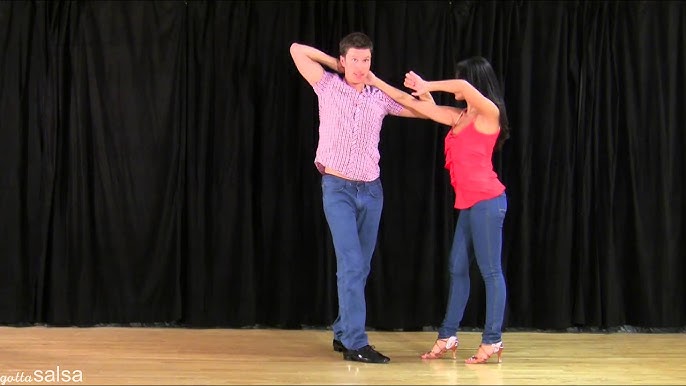In this photograph, a couple is dancing on a glossy, light brown wooden stage with a solid black pleated curtain as their backdrop. The stage is marked with elegant white overlay text in the bottom left corner that says "Goddess Salsa," with "Goddess" in cursive and "Salsa" in sans-serif. 

The man, positioned on the left, is wearing a pink, short-sleeve, button-up shirt and blue jeans with black pointed shoes. He has short brown hair and is looking to his right with a surprised expression on his face. His right arm is raised above his shoulder at an angle, while his left arm is angled downwards at his shoulder.

To his right, the woman is facing him. She has long black hair and is dressed in a pink ruffled tank top, tight blue jeans, and red high-heel shoes. Her right arm reaches behind the man's neck, and her left arm is extended out with her palm facing up.

Their synchronized dance pose highlights their graceful movements, capturing the essence of the salsa dance they appear to be performing.